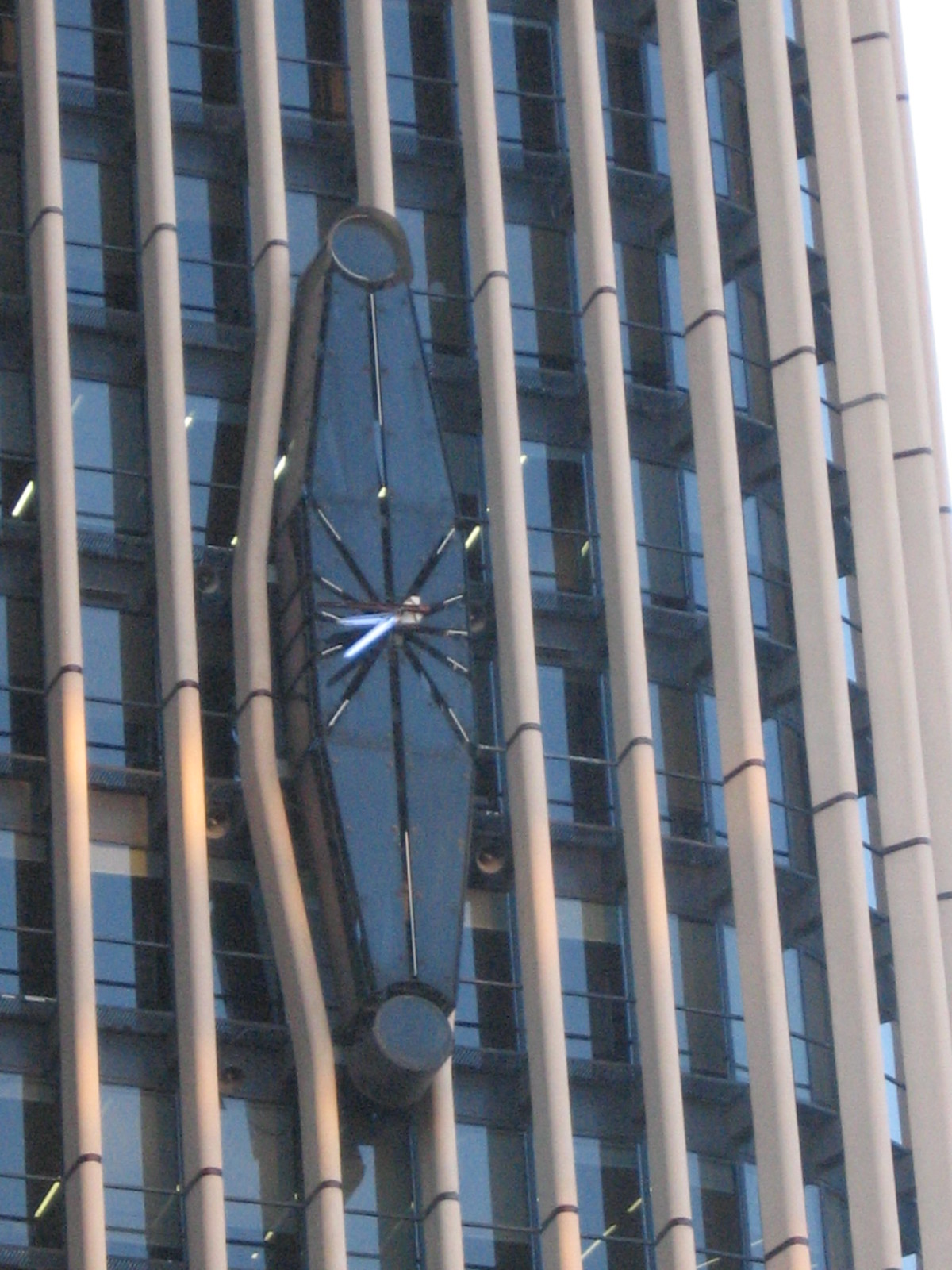A striking close-up of a modern skyscraper captured from a distant vantage point, focusing on an intriguing architectural detail. This visually captivating building is predominantly composed of sleek, reflective glass windows framed by white and tan structural beams, which add a distinctive textural element to its exterior. Central to the image is a long, slender, oblong oval structure that serves as an elegant clock. The clock face, free of numerical markings, features gold lines emanating from the center to signify the hours. Its minimalist design is complemented by finely crafted hour and minute hands in motion, adding a dynamic touch to the static architectural masterpiece.